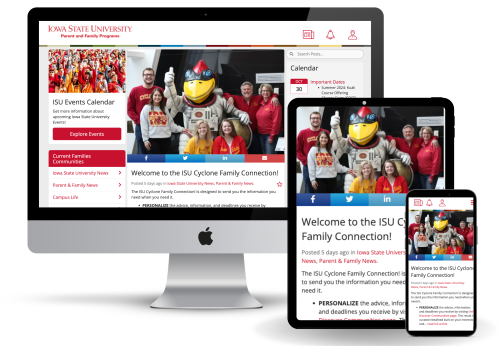A sleek iMac with a silver base and black bezels showcases the Iowa State University website on its screen. At the top, "Iowa State University" is prominently displayed in red text, accompanied by a red emblem with a bell. Below, the "ISU Events Calendar" is written in black text, followed by additional event details. On the left side of the display, there's an image of a woodpecker mascot wearing a white astronaut sweater layered over a yellow and red shirt. This mascot appears to be welcoming viewers to the "ISU Cyclone Family Connection." Further down, the text "Welcome to the ISU Family Connection" is clearly visible, indicating a recent post from five days ago in the Iowa State University Family News section. Additional personalized advice and information are mentioned, with accompanying smartphone imagery and text that is condensed in various ways.